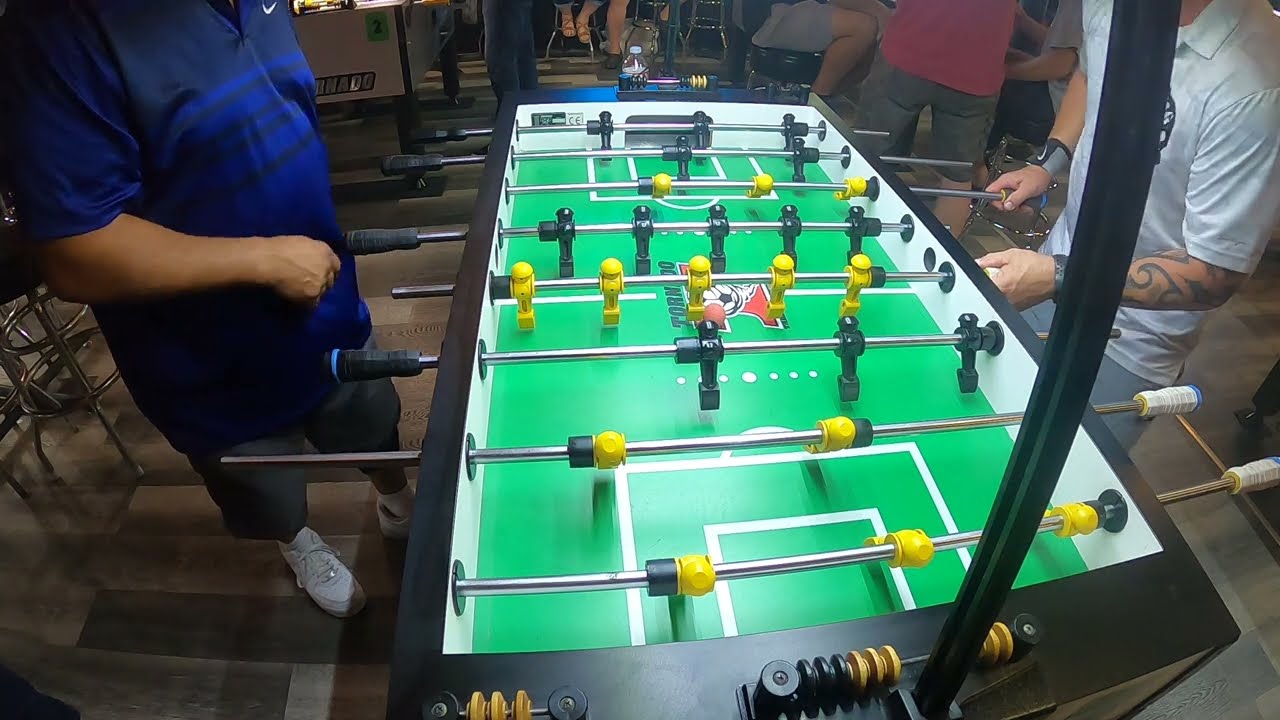In a lively bar setting with a wooden floor and scattered barstools, two men are engrossed in a game of foosball. The foosball table, illuminated from within, features a black frame, a green playing field with white lines, and gold accents on both ends. Silver poles, equipped with black rubber handles, hold black and yellow players. On the left side stands a larger man in a blue short-sleeved, navy-striped polo shirt, gray shorts, and white shoes. On the right, a thinner man with tattoos on his right forearm wears a gray polo shirt and gray shorts. Both men have their hands firmly on the handles, fully engaged in the game. Around them, other patrons can be seen sitting on barstools and mingling, adding to the vibrant atmosphere.